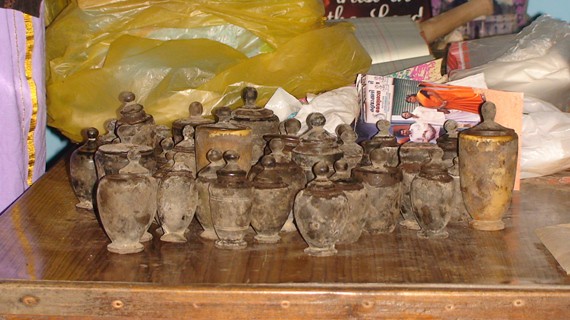The image depicts a cluttered, makeshift setup in a trashy-looking area with a sturdy, thick, dark brown wooden table at its center. The table, which has a glossy finish with dark lines running through it, is covered with a layer of white dust. Displayed on the table are numerous antique or ancient-looking urns or jugs, numbering around 30. These vessels, varying in size and shape, are primarily small and oval, with each featuring a lid adorned with a small rounded handle. The urns' exteriors are coated in brown mud, indicative of their recent excavation from an archaeological dig, though some are dusted to the point of appearing white. The majority are brown in color, while a few larger ones possess a golden hue, tarnished and almost indistinguishable from the earthy tones due to extensive wear.

Surrounding the table is a scene of disarray, with various items scattered about. Notably, there is a large, yellow plastic bag filled with plastic sheeting, along with clear white plastic bags, boxes with assorted images, cardboard tubes, large pieces of paper, and a small black sign with white lettering. Among these, there's also mention of something lavender with a yellow ribbon, a book, a notebook, and a rolling pin, adding to the chaotic mix. The setting presents a stark contrast between the dusty ancient artifacts and the clutter of modern materials, suggesting a hurried or makeshift display of the unearthed treasures.